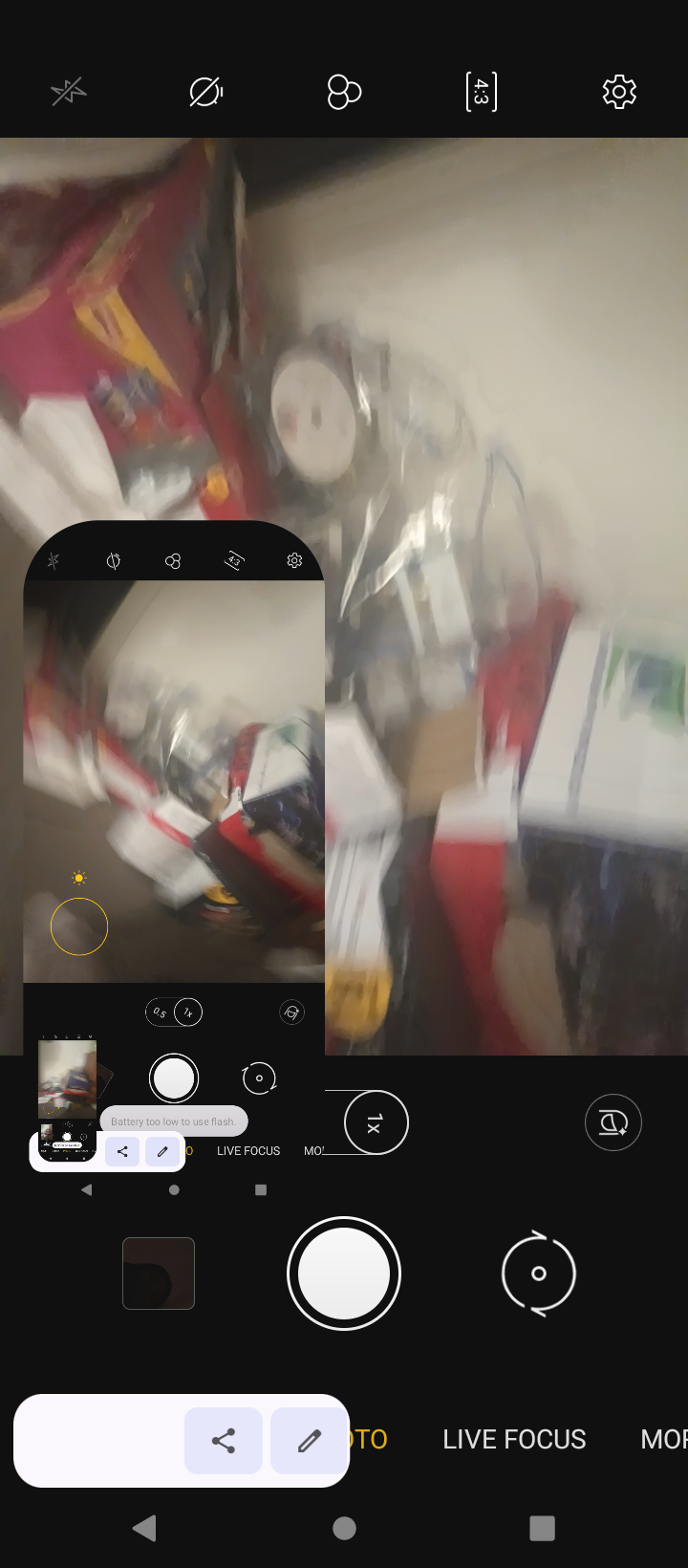This is an intricate and multi-layered screenshot captured on a smartphone, displaying a repetitive recursion of an image within an image. The primary photo appears to be taken in a cluttered space, possibly a closet or basement, featuring a white wall backdrop and an assortment of items piled up. Among the notable objects, there are visible red, yellow, and black boxes, a red and white box on the floor, and some clear plastic material, perhaps a bag. This clutter includes cardboard boxes and a yellow clock. The screenshot also reveals multiple layers of the same photo, getting progressively smaller and more distorted, adding to the visual complexity. The top part of the screenshot shows a black line, and the menu bar at the bottom of the screen displays various photo options and icons, including gear symbols for settings adjustments, a 4:3 horizontal ratio indicator, and icons for features like flash and live focus. The image is blurry, making it difficult to ascertain finer details, contributing to a sense of chaotic disarray.